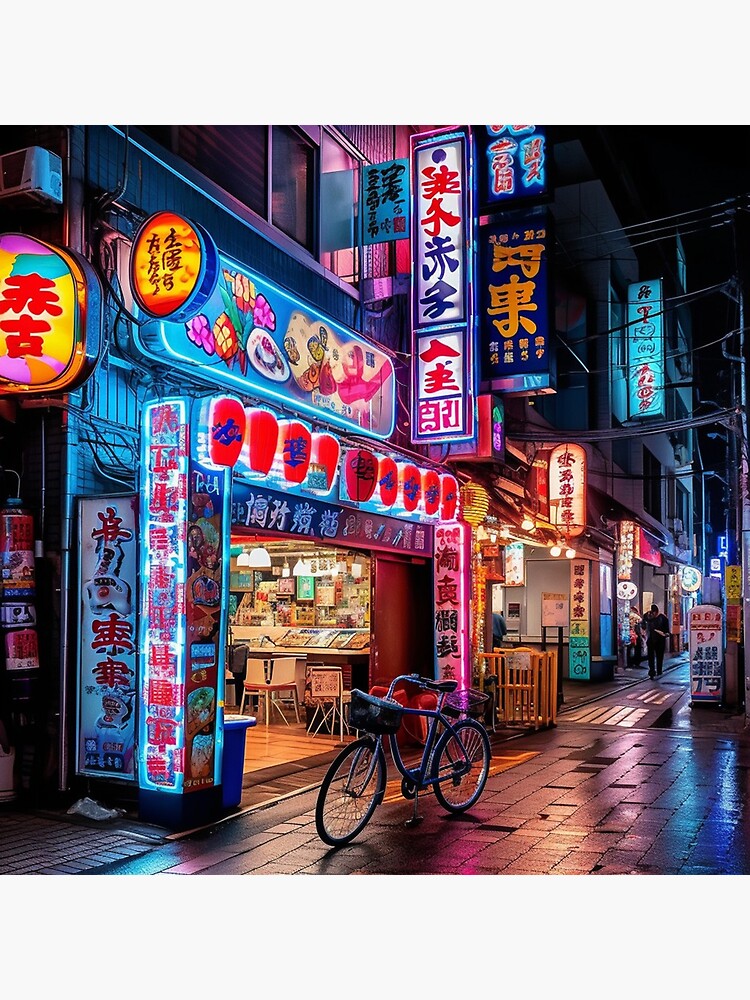The image captures a vibrant downtown area at night, likely in China, Japan, or Korea. The scene is adorned with a plethora of brightly lit neon signs featuring an array of colorful characters, primarily in red, blue, yellow, orange, pink, purple, and turquoise. The urban landscape is bustling with illuminated storefronts, creating a dynamic visual reminiscent of a busy business district or even Las Vegas. In the foreground, a solitary bicycle is parked, implying its owner has ventured into a nearby establishment, which could be a restaurant or perhaps an art show given the eclectic mix of lights and textures. The ground glistens with rainwater, reflecting the vivid array of neon lights, adding to the night-time beauty of the scene. The street appears surprisingly quiet, devoid of people, enhancing the focus on the neon-lit environment and the tranquil, rain-soaked street.